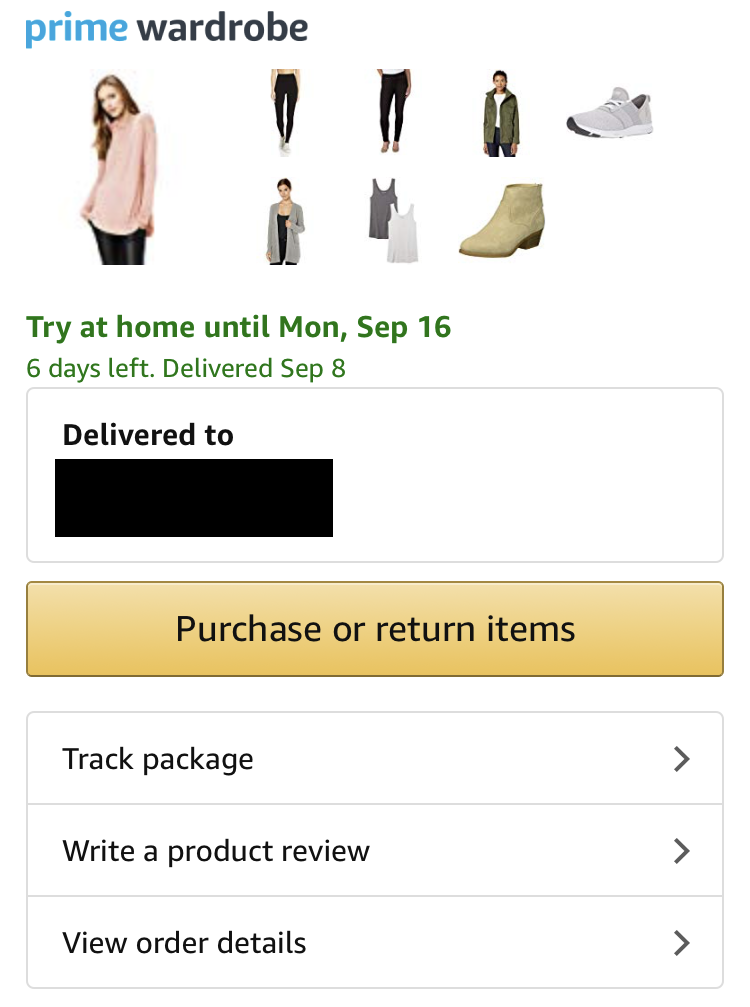This is a detailed screenshot taken from the Amazon Prime Wardrobe section within the Amazon shopping app. At the top left corner, the text "Prime Wardrobe" is prominently displayed. Below this header, there's a gallery showcasing various clothing items available for purchase. The first item in the list features a woman modeling a pink top, followed by images of two different people wearing black sweatpants or leggings. Next, there's an individual posing in a green jacket, followed by a shoe, and another woman modeling a long grey cardigan. Further down, two camisoles are displayed along with a single boot.

Beneath the item images, green text informs the user that they can "try at home until Monday, September 16" with "six days left" to return items, noting the delivery date of "September 8." There is a small window indicating the delivery address, which is blacked out for privacy. Below this, a prominent yellow button allows the user to "Purchase or return items."

At the bottom of the screen, there is another section with three options: "Track package," "Write a product review," and "View order details." The entire screenshot features a clean, white background for clarity and ease of use.